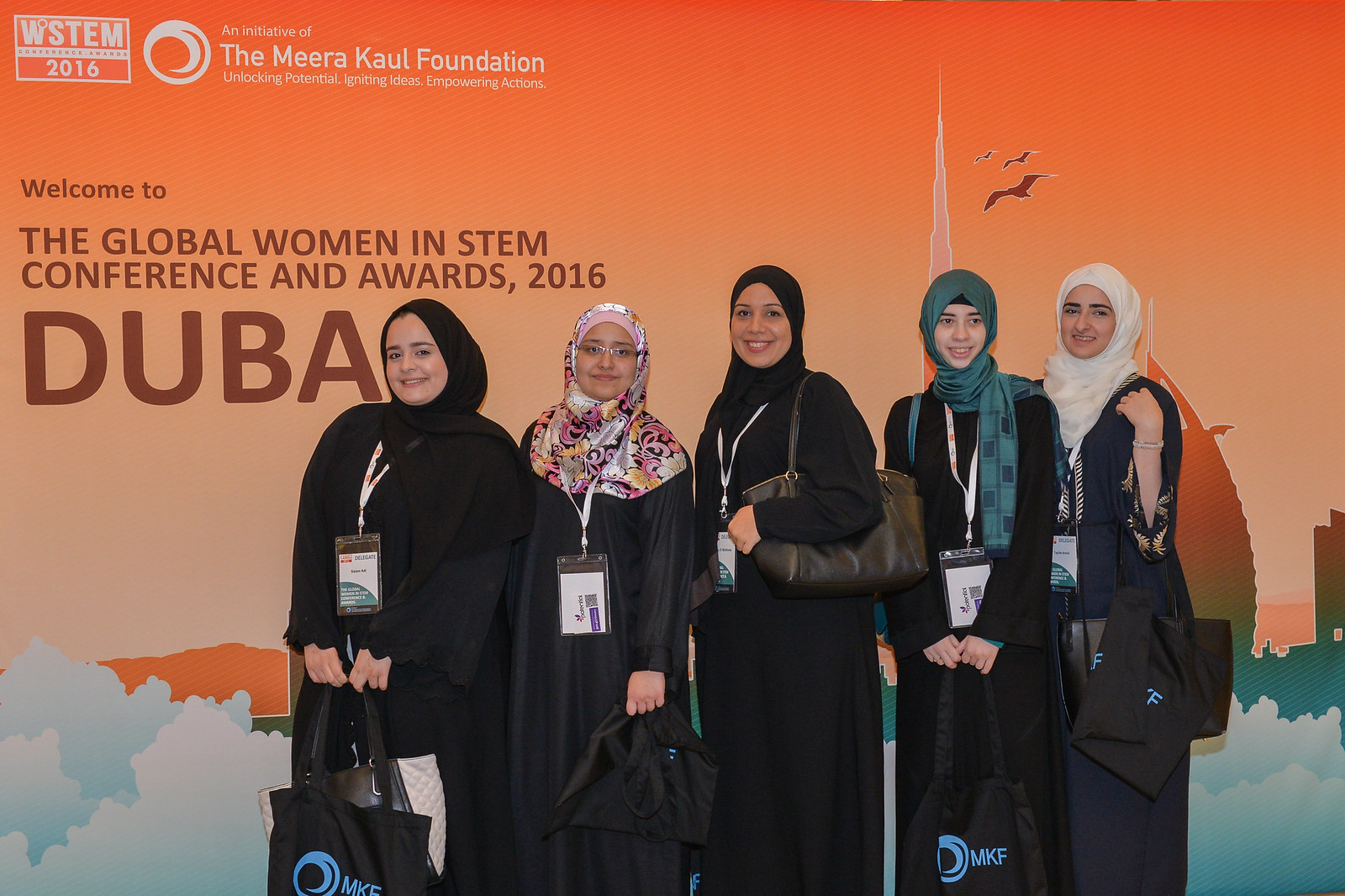Five women, dressed in black burqas and hijabs, stand in a semi-line in front of a large poster. The first woman, entirely in black, holds two bags—one marked with the blue logo "MKF." The second woman wears glasses and has a vibrant, multi-colored floral headscarf, contrasting with her black ensemble. Behind her, the third woman wears a black burqa with a dark bag over her shoulder. The fourth woman sports a green headscarf adorned with dark rectangles, coupled with a black dress and a bag. The fifth woman, in a dark navy blue dress, accessorizes with a white headscarf and another bag bearing the same "MKF" logo. All have lanyards with ID badges around their necks.

The backdrop features a towering poster with an orange gradient, transitioning to blue at the bottom, with wispy clouds and a depiction of the Dubai skyline, including the Burj Khalifa and flying birds. Text on the poster reads: "Welcome to the Global Women in STEM Conference and Awards 2016, Dubai," complemented by the logos "WSTM 2016" and a circular emblem. The poster also mentions, "An initiative of the Miracle Foundation. Unlocking potential, igniting ideas, empowering actions."